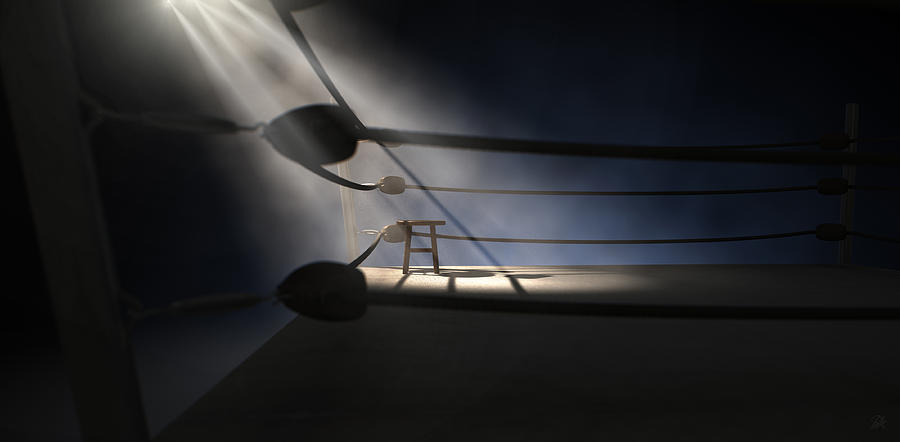This indoor picture is enveloped in darkness, with an overarching dim theme. The scene centers around a boxing ring, identifiable by the corner pads and enclosing ropes. Despite the murkiness, a stream of light pierces through from the top, creating a slightly smoky atmosphere accentuated by this beam. The most striking detail in this shadowy setting is a wooden stool placed in one corner of the ring, dramatically highlighted by a spotlight, drawing attention to its prominent position amidst the gloom.